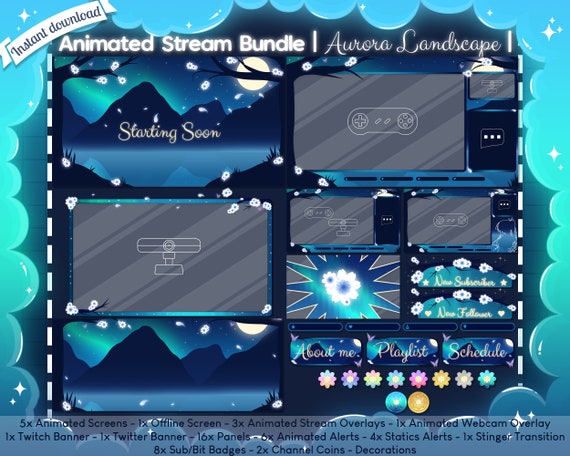The image showcases a detailed and vibrant compilation of various graphics under the headline "Animated Stream Bundle - Aurora Landscape." The collection is presented with a bubbly aqua frame and a serene winter-themed color scheme, featuring shades of blue, white, and teal. 

At the top, a white banner reads "Instant Download." Below it, the main section divides into several boxes displaying different components of the bundle. Notably, a deep blue mountainscape with a neon sky overlay carries "Starting Soon" in script. Another box features a gray background with a video game controller icon, while another includes an empty screen with a webcam overlay. 

Further down, smaller boxes contain labels such as "New Subscriber," "New Follower," and a row of three boxes titled "About Me," "Playlist," and "Schedule." Alongside these visuals are lists detailing the bundle's contents: five animated screens, one offline screen, three animated stream overlays, one animated webcam overlay, one Twitch banner, one Twitter banner, 16 panels, six animated alerts, four static alerts, one stinger transition, eight sub/bit badges, two channel points icons, and various decorations. 

This creative and technologically integrated compilation image captures the essence of a visually appealing and organized streaming bundle, perfect for a calming and engaging winter-themed stream setup.